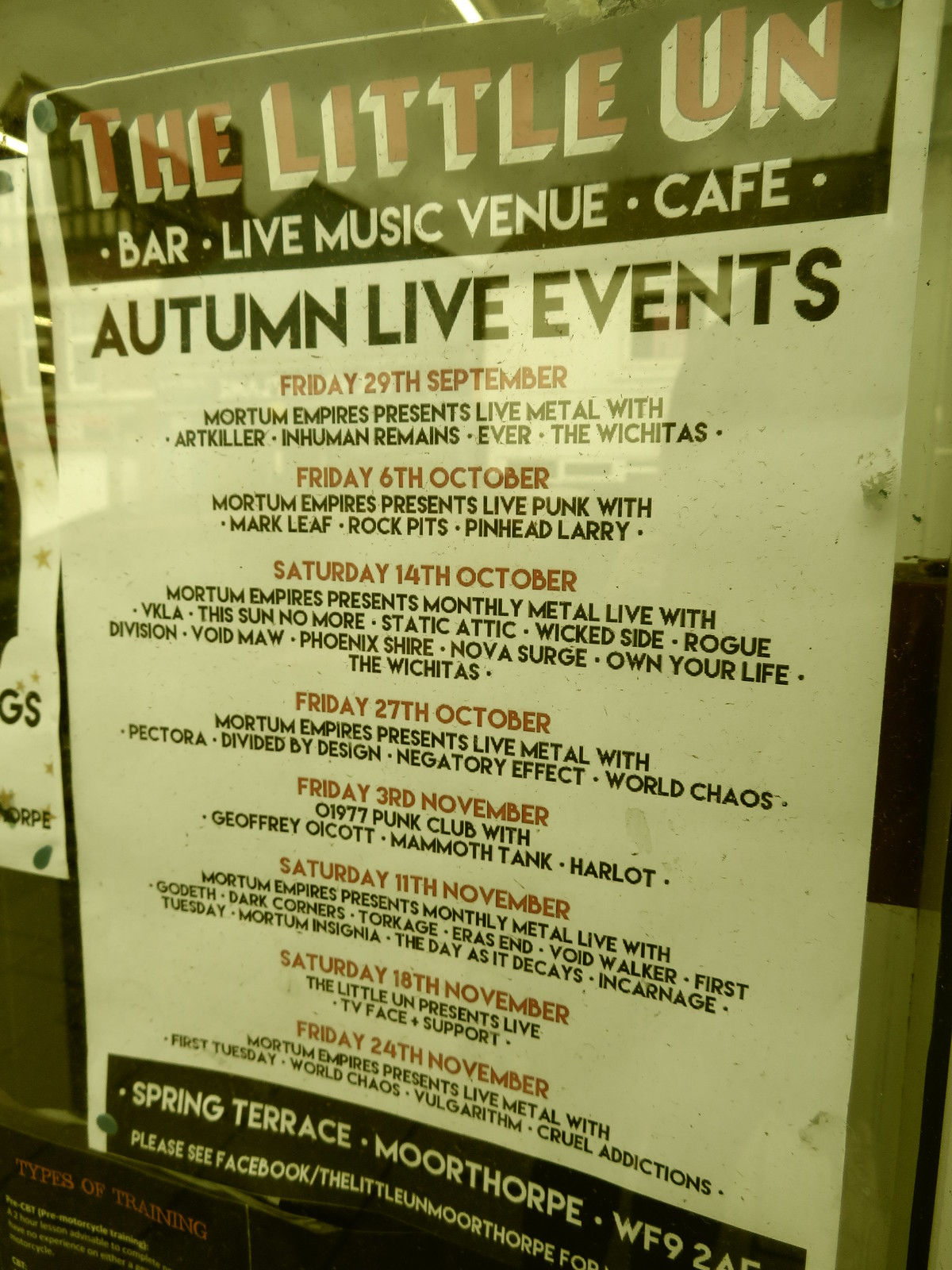This image depicts a rectangular poster attached to a wall and positioned behind a transparent glass window, advertising a bar and cafe known as "The Little UN." The poster's title, encapsulated in a black box with "The Little UN" written in red, announces it as a bar, live music venue, and cafe. Below this, in white, are the words "Autumn Live Events." The events are detailed with specific dates: 

- Friday, 29th September: Mortem Empires presents live metal with Art Killer, Inhuman Remains, Ever, and The Witch It As.
- Friday, 6th October: Mortem Empires presents live punk with Mark Leaf, Rock Pits, and Pinhead Larry.
- Saturday, 14th October: Additional bands are listed.

The poster features a white background and lists a total of eight dates with their respective events. At the bottom, the location is indicated as "Spring Paris, Moor Thorpe, WF92." Surrounding the main poster are glimpses of other posters on the same wall, adding to the venue's promotional material.